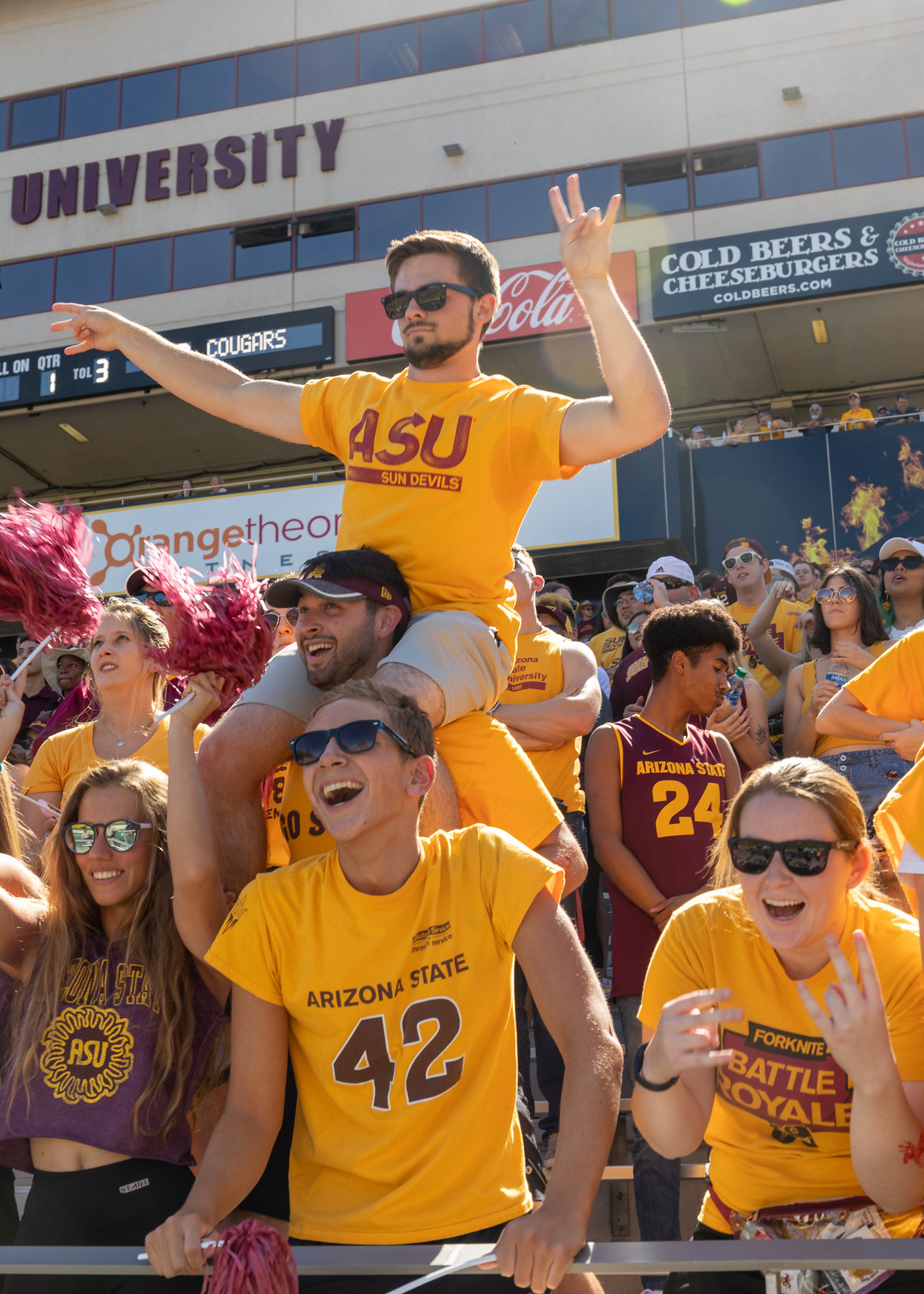This outdoor photograph captures the lively atmosphere of a college sporting event at a stadium, packed with enthusiastic Arizona State University (ASU) fans. Central to the image is a diverse group of young people, primarily students, who embody the energetic spirit of the event. 

In the foreground, prominently featured is a young man with blonde hair, dressed in a yellow ASU t-shirt with the number 42 emblazoned on it, gripping a railing while smiling broadly, his eyes hidden behind a pair of sunglasses. To his left stands a young woman with long light brown hair, also wearing sunglasses. She is dressed in a purple t-shirt that reveals her midriff and black pants, her cheerful demeanor framed by her bright smile. 

To his right, another young woman leans forward; she has blonde hair pulled back and wears sunglasses, sporting a yellow t-shirt with "Battle Royale" printed across the front.

Directly behind this group, another man wearing a yellow t-shirt and a visor lifts a fellow fan onto his shoulders. This elevated fan, donned in a yellow ASU shirt, sunglasses, and sporting a beard and mustache, jubilantly raises his arms—one extended outward and the other bent with a fist towards the sky.

In the background, the crowd fills the stands, with a visible scoreboard displaying advertisements for "cold beers and cheeseburgers," and banners including one for Coca-Cola. The facade of the stadium includes partially visible text reading “University,” and beneath, there appear to be skyboxes or press levels.

Overall, this image vividly illustrates the fervor and communal joy of the ASU fans at the stadium, highlighting key individuals and the collective atmosphere of the event.